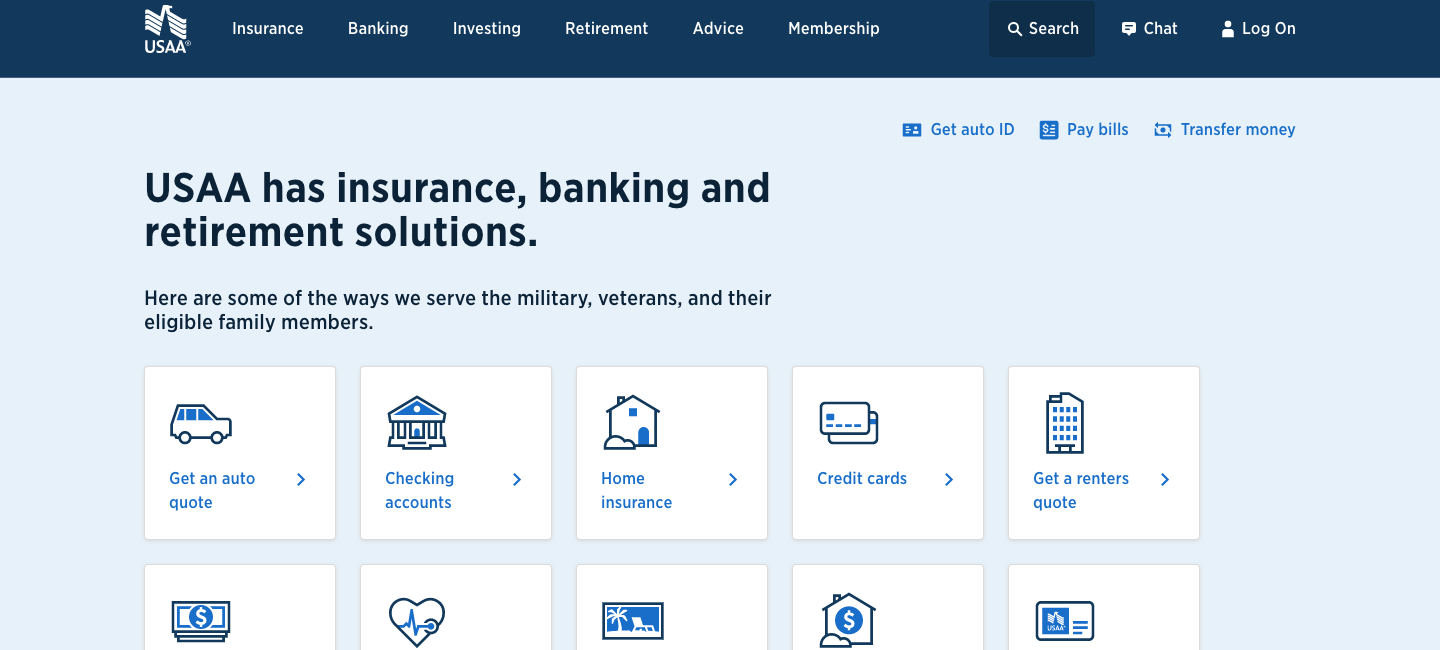This is a screenshot of the USAA website. In the upper left-hand corner, the recognizable white USAA logo is displayed against a navy blue header bar. The header bar extends across the top of the page and includes various navigation options: Insurance, Banking, Investing, Retirement, Advice, Membership, Search, Chat, and Logon.

Beneath the header bar, the background transitions to a light blue or baby blue color. Prominently displayed in dark navy blue text is a header stating, "USAA has insurance, banking, and retirement solutions." Below this, there is a subheading that reads, "Here are some of the ways we serve the military veterans and their eligible family members."

Following this introduction, several clickable cards are presented, offering different services. These include:
- "Get an Auto Quote"
- "Checking Accounts"
- "Home Insurance"
- "Credit Cards"
- "Get a Renter's Quote"

Additionally, there is another row of cards underneath, though only the icons are visible as the text is cut off in the screenshot.